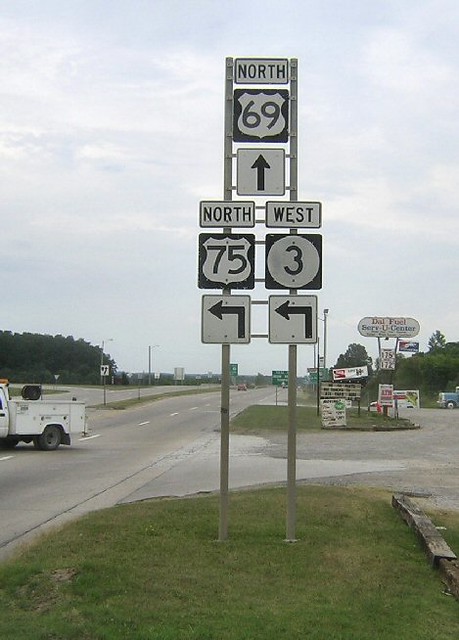This image captures a busy intersection featuring multiple traffic signs and a part of a gas station. The central traffic sign displays an array of directional indicators: the primary sign shows "North 69" with an upward-pointing black arrow. Below it, there are two additional signs - "North 75" with a left-pointing arrow and "West 3," also directing left. These signs are mounted on metal stakes placed on a grassy area. In the background, a white utility or pickup truck is visible on the highway. The road appears to have two lanes in one direction and possibly two or three lanes in the opposite direction. The gas station on the corner is identified as "Dell (or Dow) Fuel Serv-U Center," featuring a gravel driveway and an older blue truck parked nearby. There is a small billboard at the station, indicating gas prices at $1.75 or $1.25, suggesting that the image might be from an earlier time period. Additionally, there are green traffic signs in the distance, although their details are not discernible.